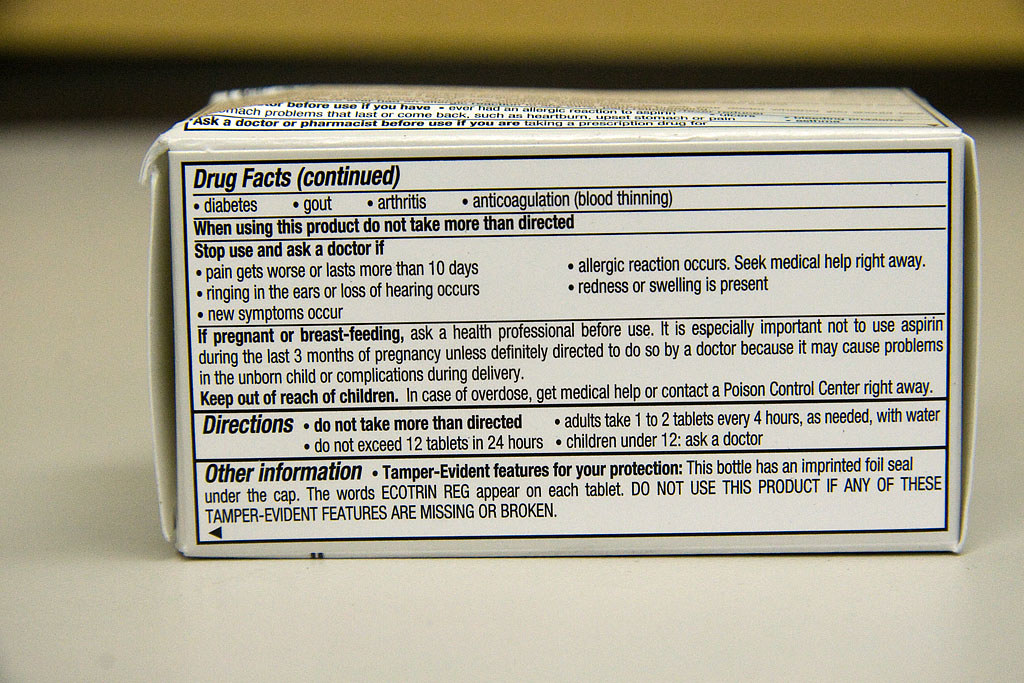This real-life photograph showcases the side of a medicine product packaging prominently labeled "Drug Facts Continued" in bold black text. Below this heading, the packaging lists specific conditions and medications including diabetes, gout, arthritis, and anticoagulation (blood thinning). Further down, advisory text warns users, "When using this product, do not take more than directed." It also advises to "Stop use and ask a doctor if pain gets worse or lasts more than 10 days, ringing in the ears or loss of hearing occurs, new symptoms emerge, an allergic reaction occurs (seek medical help right away), or redness or swelling is present."

Additional guidance includes, "If pregnant or breastfeeding, ask a health professional before use."
The text continues with sections detailing directions and other important information. The packaging is set against a white surface, with a blurry backdrop featuring indistinct black and yellow lines, indicating that the camera's focus is intentionally directed towards the product packaging.